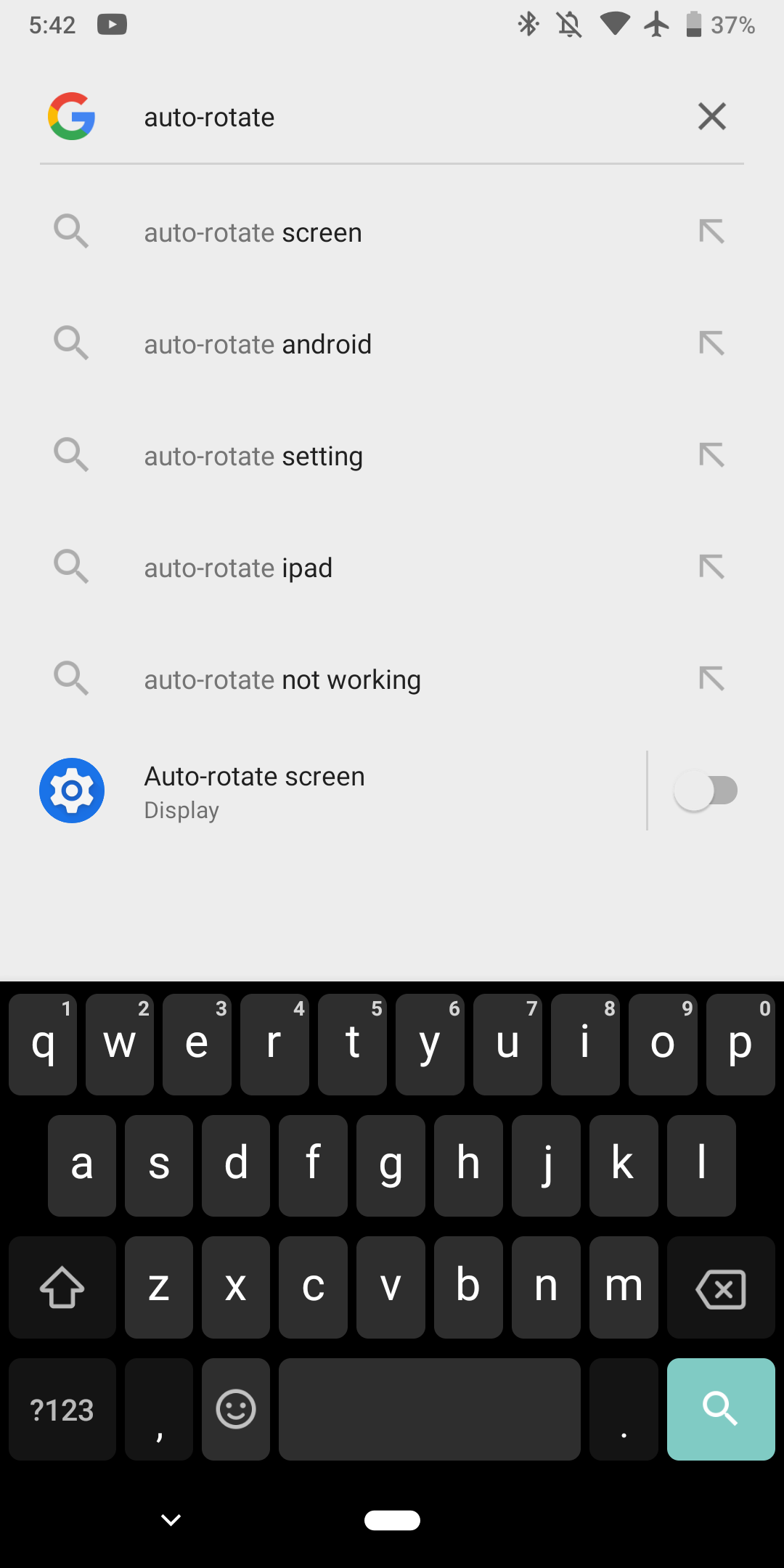The screenshot captures an Android phone settings page with a search term entry of "auto-rotate." 

The top left corner displays a gray background with the time indicated as 5:42. Adjacent to the time in the top right corner, various status icons appear, including Bluetooth, airplane mode, and a battery symbol showing 37% charge. 

Just below these icons, the Google search bar is positioned, displaying the typed search term "auto-rotate." To the right of this search term is an 'X' icon, likely for clearing the search entry. 

Directly underneath the search bar, several search suggestions are listed:
- A magnifying glass icon followed by "auto-rotate screen."
- Another magnifying glass icon with the text "auto-rotate Android."
- A third magnifying glass icon next to "auto-rotate setting."
- Yet another magnifying glass icon with "auto-rotate iPad."
- A fifth magnifying glass icon paired with "auto-rotate not working."

Following these suggestions, there is a blue circle containing a gear icon labeled "auto-rotate screen display," with an adjacent option that is currently disabled.

At the bottom of the screenshot, the alphanumeric keyboard is displayed against a black background. The bottom row of the keyboard includes a key combining the question mark and numerical access (1, 2, 3), a comma key, a smiley face icon, the space bar, a period, and a blue key on the far right bearing a white magnifying glass icon.

This detailed visual information points to the user navigating their settings to address or adjust the "auto-rotate" function on their Android device.